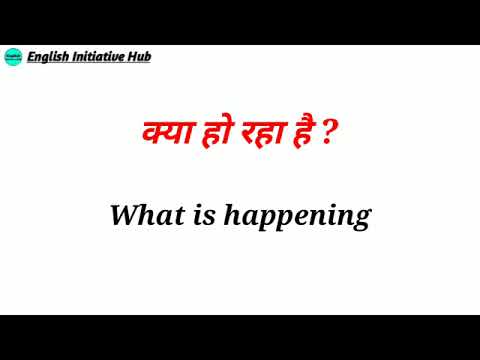This wide rectangular image appears to be a screenshot of a slide or video, featuring black strips at the top and bottom that partially crop the frame. The background is entirely white. In the top left corner, there is a turquoise circle with two blue horizontal lines passing through it. Next to it, an underlined, bold, italicized black text reads "English Initiative Hub." Dominating the middle of the image is a thick red question written in a foreign language that could be either Asian or Russian; this question concludes with a red question mark. Below the red question, in bold italicized black font, it reads "what is happening." The positioning and context suggest that the red characters may be a translation of the English text.